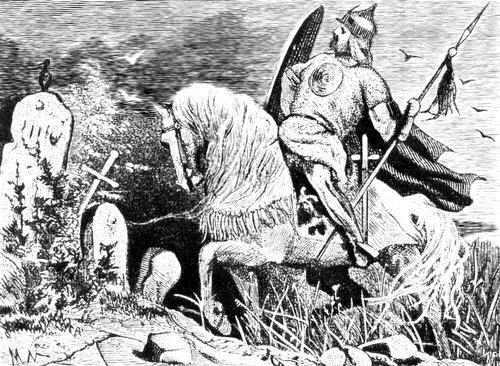This black-and-white image, reminiscent of a vintage engraving, depicts a warrior in mid-battle on horseback. The central figure is a man sitting on a horse, both facing left. The warrior is armored with a helmet adorned with a pointy top and a scarf hanging beneath it, a circular breastplate, and chainmail partially visible beneath his cloak that billows behind him. His right hand grips a spear adorned with a tassel, while a large shield is positioned in front of him, and a sword hangs at his side. The horse appears to be in mid-stride, suggesting movement towards the left. 

In the foreground to the left of the horse, partially obscured by brush and grass, are multiple grave markers or gravestones, along with a cross planted in the ground, casting some ambiguity as to whether it might be a sword or a grave marker. The background reveals a sky filled with shades of gray, adding to the somber tone of the scene. On the right side of the image, four birds can be seen in flight, contributing to the overall sense of motion and atmosphere.